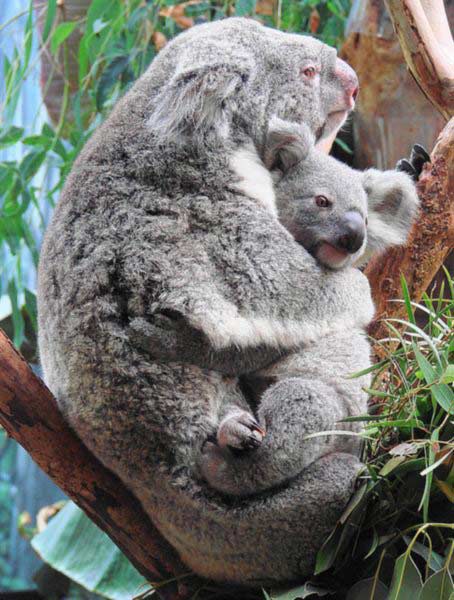In the image, we see a mother and baby koala nestled together in the crook of a tree, which appears to be a eucalyptus. The mother koala, identifiable by her pinkish nose, is firmly holding her baby against her chest as she clings to the side of the medium brown tree trunk. The baby, with a distinct black nose and an adorably pudgy face, peeks over her shoulder, looking downward with curious eyes. Surrounding them are tree leaves and some vines, contributing to the natural ambiance. The photograph is fairly zoomed in, emphasizing the intimate moment between the two koalas, while a blue wall or rock face is faintly visible in the background, hinting that this scene might be set within an enclosure at a zoo or sanctuary rather than in the wild.